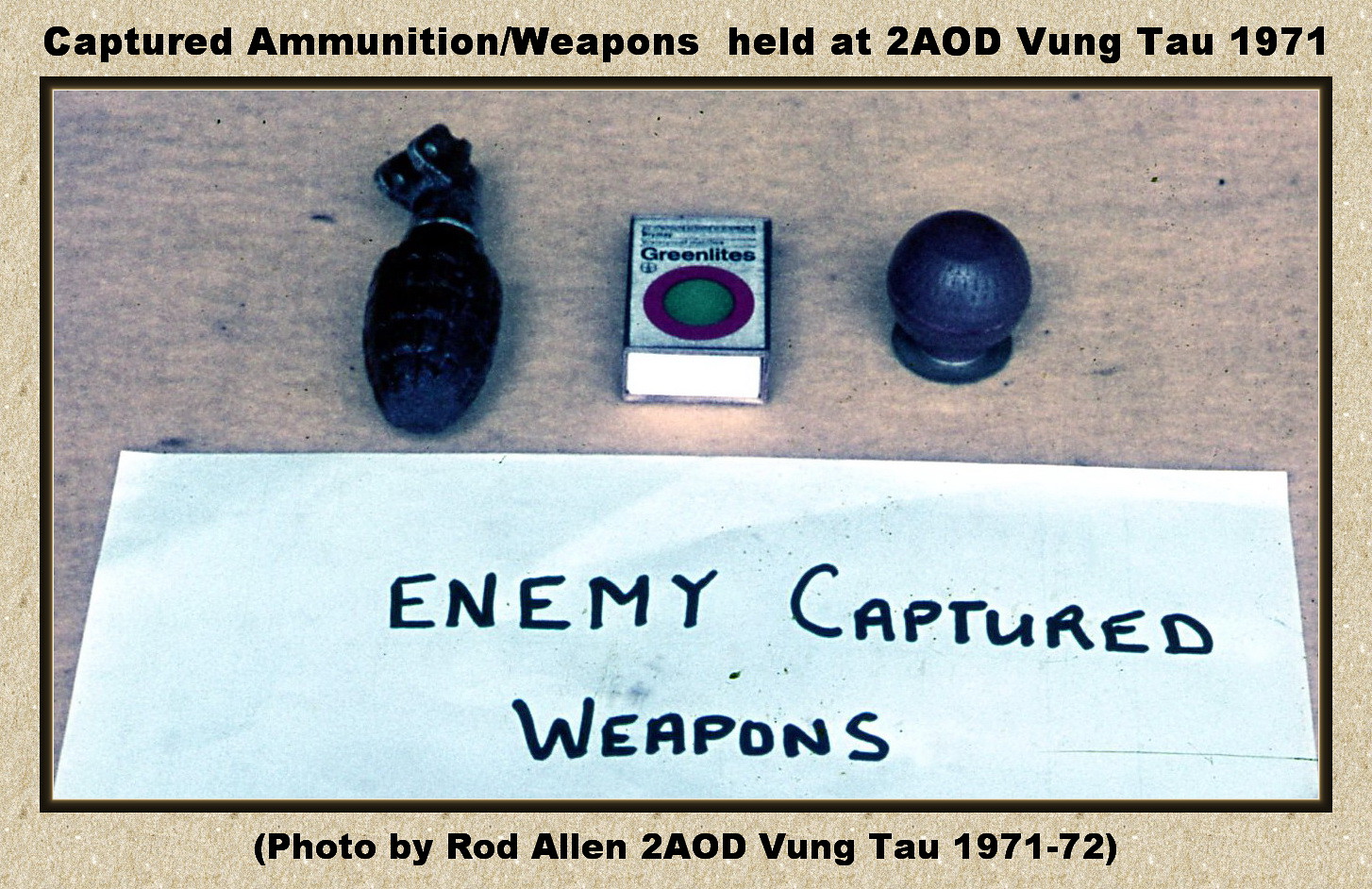In this detailed image, the photograph is framed by a tan, cream, or beige border with a very thin, dark brown edge. The top of the border is inscribed in black text, reading, "Captured Ammunitions/Weapons Held at 2 AOD Vung Tau, 1971," with "Photo by Rod Allen, 2 AOD Vung Tau, 1971-72" beneath it.

The central focus of the image is a collection of enemy-captured weapons, neatly positioned at the center of a gray stone surface, likely a table. Prominent among these weapons are several grenades. To the left is a black hand grenade without its pin, suggesting it could be dangerous. In the middle is an object featuring a red circle with a green circle at its center, labeled "green lights"—its exact nature unclear. Additionally, another black, circular grenade is visible.

Below the weapons, a rectangular white piece of paper displays the handwritten text, "Enemy Captured Weapons," written in all caps, possibly with a Sharpie. The setting suggests the possibility of being either indoors or outdoors, likely in Vietnam, as indicated by the references to Vung Tau, a known location during the Vietnam War. The colors in the image include shades of tan, black, gray, purple, and green.